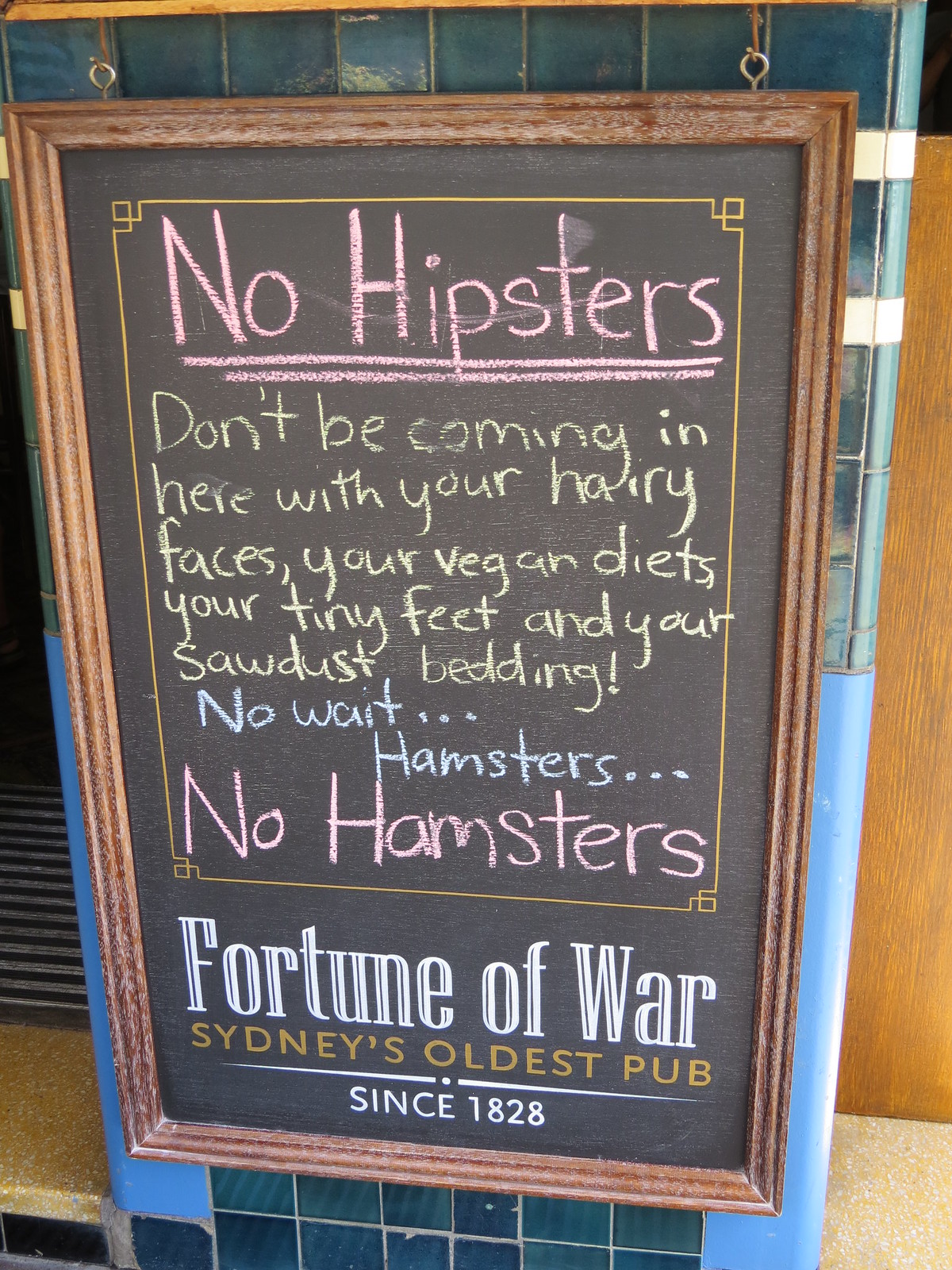The photograph is taken outdoors during the daytime, featuring a rectangular, blue-tiled column with a hanging chalkboard sign. The chalkboard, encased in a brown wooden frame, is the focal point of the image. At the top, written in pink chalk and underlined twice, it reads, "No hipsters." Below that, in yellow chalk, it humorously warns, "Don't be coming in here with your hairy faces, your vegan diets, your tiny feet, and your sawdust bedding!" This is followed by a message in blue chalk stating, "No wait ... hamsters ..." and then in bold pink chalk, "No hamsters." Towards the bottom of the chalkboard, in white print, it declares "Fortune of War," and underneath that in gold print, it proudly notes, "Sydney's oldest pub." Centered at the very bottom in white, it states, "Since 1828."